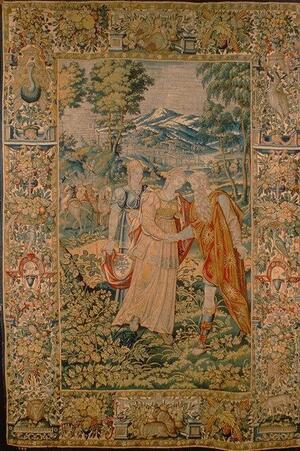This image captures a vintage tapestry with muted, faded colors, suggesting age and delicacy, possibly several centuries old. The central scene, framed by a detailed rectangular border with small, indistinct floral designs, features three main figures. At the center, a man with a beard, dressed in a flowing orange robe, extends his hand in greeting to a woman in a long peach gown. Behind them to the left stands another figure, also dressed in elegant attire, holding a basket of flowers. Surrounding the trio is a picturesque garden with lush green foliage, while the background reveals a tranquil landscape with trees and distant snow-capped mountains under an expansive sky.